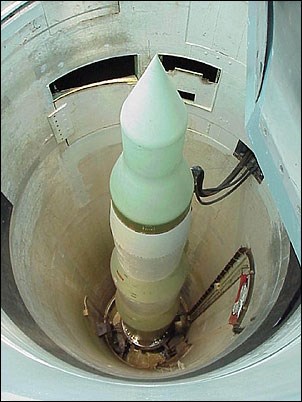This detailed photograph, presented in a portrait layout with a thin black border, captures the internal view of a cylindrical structure, likely part of a military or aerospace vehicle. At the center of the image, a long, rocket-like object is prominently featured. This object has a white body with a green tip, and it tapers to a sharp point. The cylindrical structure housing the rocket is either white or silver, difficult to distinguish in the lighting. Wires, predominantly black, extend from the top of the rocket and run along the inner walls of the cylinder, which appear to be concrete. Additionally, there's a silver base at the bottom of the cylinder. Surrounding the rocket and wires, there's an open door with additional wiring. While the exact scale of the rocket and cylinder is ambiguous, no people or text are present in this photograph, providing an unobstructed view into this technologically complex setting.